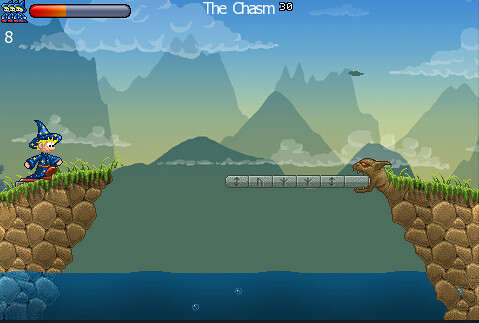In this video game scene displayed on the screen, the top of the image features the title "The Chasm" in white text, accompanied by the number "30". The background showcases a majestic mountain range that stretches upward into the sky, with white clouds scattered above. In the foreground runs a blue river or stream, adding a serene yet dynamic element to the landscape. On the left side of the stream, a stone hill covered in vibrant green grass ascends, upon which stands a small, intriguing character. This character appears to be a wizard, donned in a blue robe adorned with gold stars, and a matching wizard hat. His blonde hair peeks out from under the hat, and his wide-eyed expression suggests a mix of curiosity and surprise. Opposite the wizard, on the other side of the stream, is a formidable brown dog. This fierce creature has red eyes, pointy ears, and is baring his sharp fangs, with his mouth open to reveal an object he is gripping firmly. The tension between the characters adds an exhilarating edge to the picturesque scene.